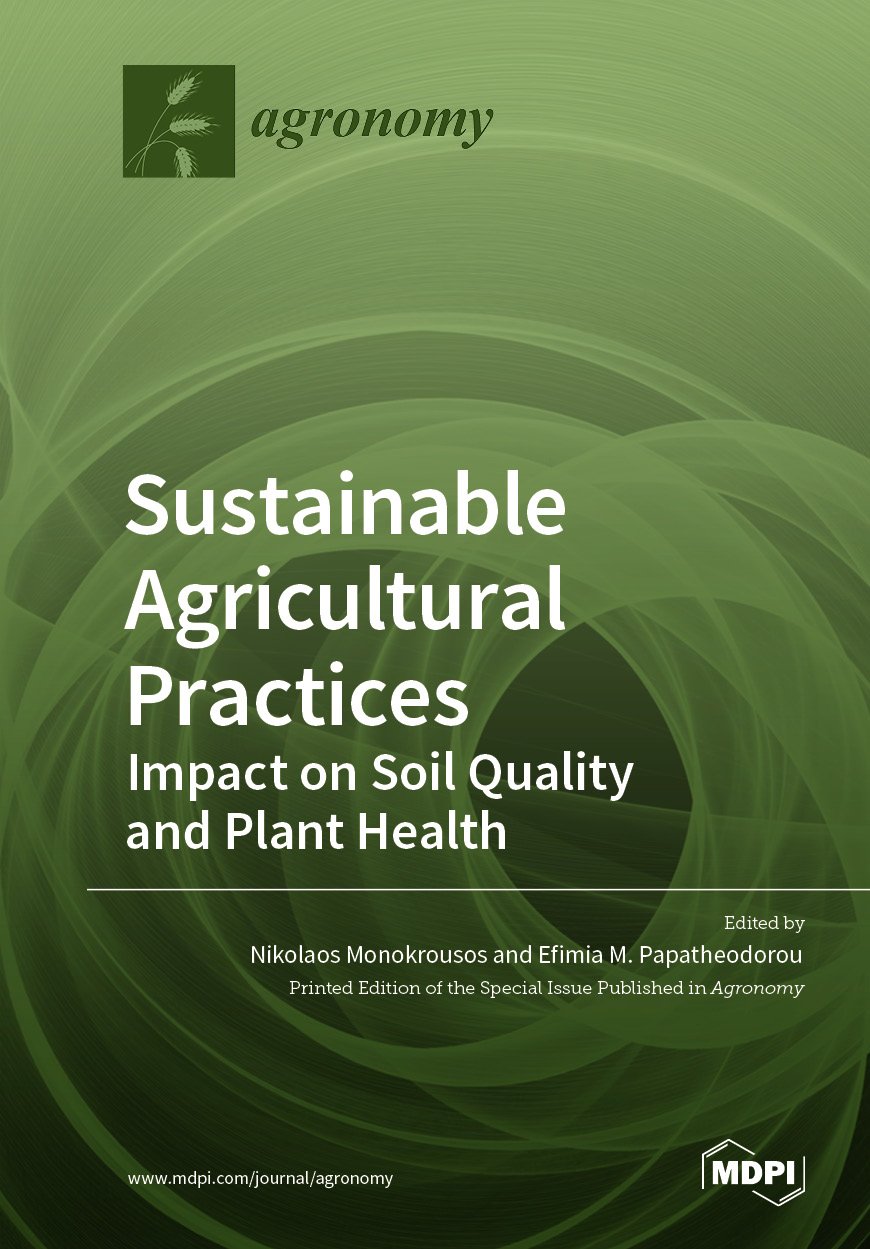The image is a rectangular flyer or pamphlet, approximately five to six inches high and four inches wide, predominantly featuring various shades of green. It has an abstract, swirling pattern created by concentric circles that transition from green to white. In the upper left-hand corner, there is a small dark green square containing a light green illustration of three strands of wheat. To the right of this square is the word "AGRONOMY" written in dark green print.

Centrally positioned on the flyer is a block of text in large white letters that reads "SUSTAINABLE AGRICULTURAL PRACTICES." Below this are two slightly smaller white lines of text stating "Impact on Soil Quality and Plant Health," underlined by a white horizontal line. Further down, in small white print, it reads "Edited by Nicholas Monacrosis and Ephemia M. Papatheodoro, printed edition of the special issue published in Agronomy." 

In the lower left-hand corner, the URL "www.mdpi.com/journal/agronomy" is printed in white. The lower right-hand corner features the logo "MDPI" in large white print.